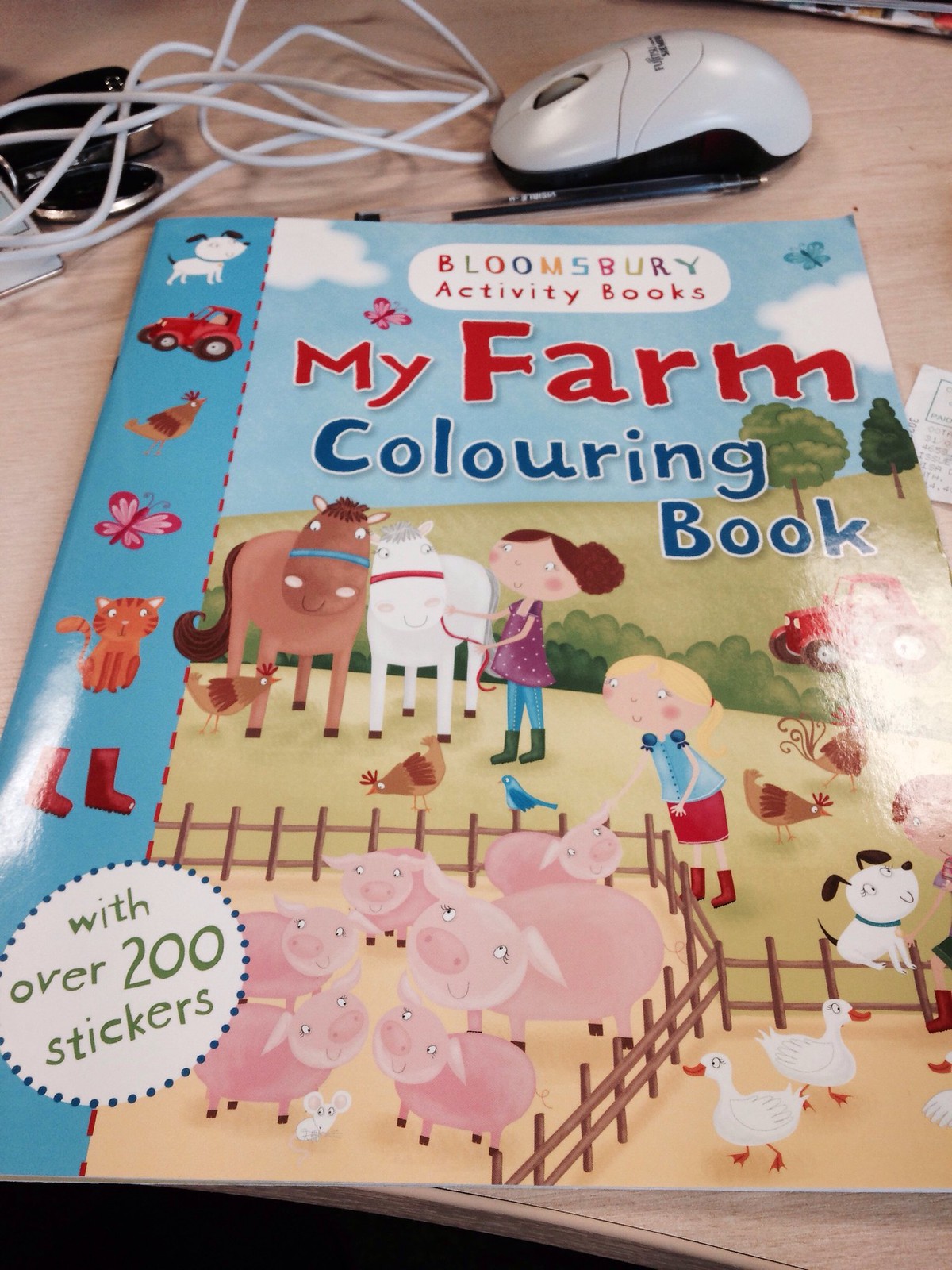The image showcases a children's coloring book titled "My Farm Coloring Book" from Bloomsbury Activity Books, prominently positioned on a light tan wooden desk. The book's cover features vibrant illustrations meant to appeal to young children, such as cheerful kids and animals in a farm setting. Notable characters include a girl with brown hair tied back in a bun, dressed in a purple top, blue jeans, and green boots, tending to a brown and a white horse; and a blonde girl with a blue blouse, red skirt, and red boots, petting pink pigs. Additionally, there is a cropped image of a child playing with a dog in the bottom right corner. Surrounding these figures, the scene is filled with other farm animals like chickens, ducks, and pigs, contributing to the lively farm atmosphere. The book also promises "over 200 stickers," as indicated by a white circle with green lettering on the cover. Adjacent to the book on the desk are a white computer mouse with a bunched-up cord, a pen, and some indistinct items—possibly a pendant, a lighter, or batteries—nestled under the cord, all contributing to the everyday desktop clutter.